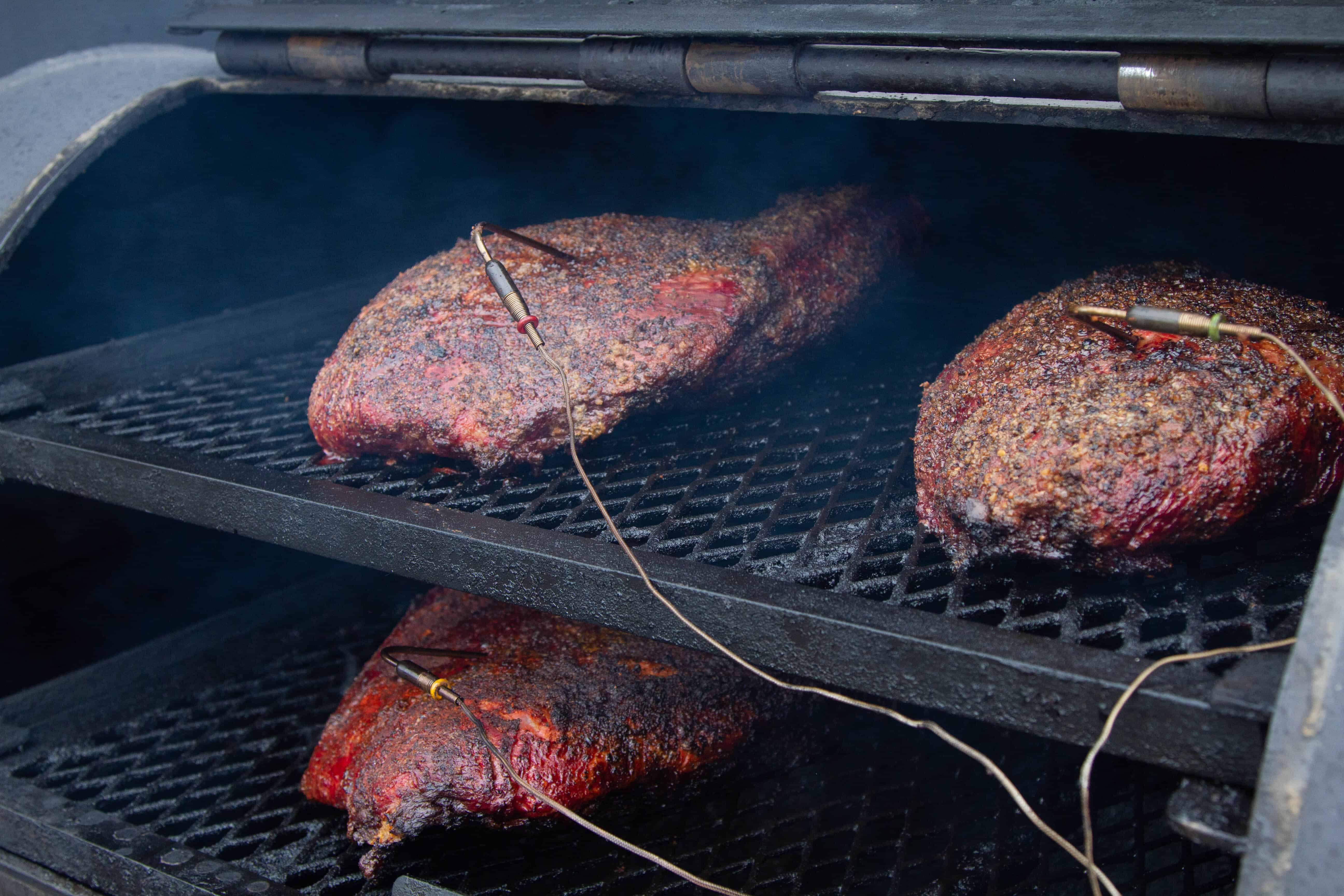In this detailed, close-up image of an outdoor scene, a grill or smoker is shown with two shelves laden with pieces of meat, possibly hams, roasts, or ribs, being cooked or smoked. The well-worn blackened grill features heavy gauge, diamond-shaped metal grates that form the two levels. On the bottom rack, where active cooking is likely occurring, one piece of meat is notably charred with some red areas, and a thermometer wire inserted to ensure precise temperature control. Similarly, the top rack, likely a warming rack, holds two other pieces of meat, each pierced with a rod connected to copper-colored wires, again to monitor their temperature. The grill’s front is hinged open, revealing the interior and focusing the viewer’s attention on the cooking process. Smoke pervades the scene, indicating ongoing cooking, albeit without visible flames. The wires presumably lead to a digital readout outside the frame, ensuring each meat piece is cooked to perfection.